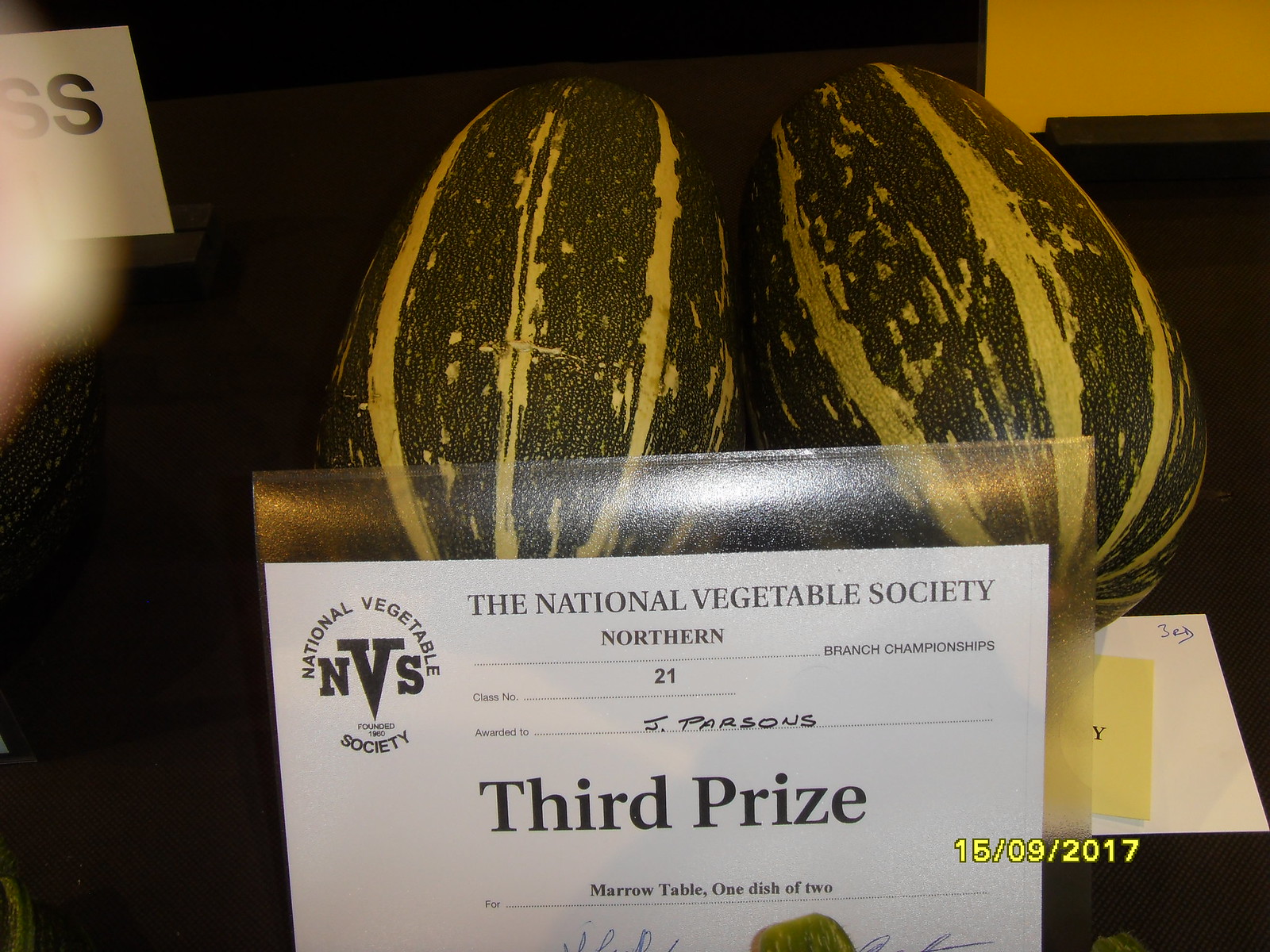In this horizontal-rectangular color photograph, taken on 15-09-2017, a prize-winning entry is showcased from the National Vegetable Society's Northern Branch Championships. The central focus is a white certificate card prominently positioned in the foreground, which announces a third prize awarded to Jay Parsons for his entry in class number 21, "Marrow Table, one dish of two." The card features black text and includes the National Vegetable Society (NVS) logo in its top left corner. Behind the certificate, two enormous green squash with yellow stripes, which might initially be mistaken for watermelons, sit side by side on a dark-colored table. These squash are the prized vegetables. In the right lower corner of the image, there is a small piece of paper, presumably detailing the squash's variety and cultivation information. The background features additional subdued elements, including another black plate and a white wall, which add context but do not detract from the central prize-winning display.